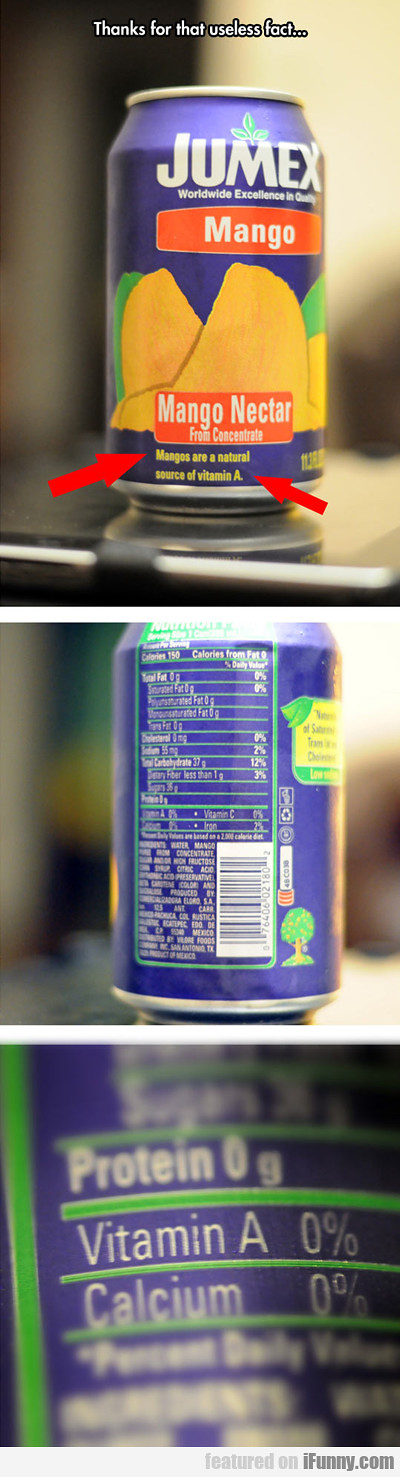The image is a collage of three photos vertically arranged, each depicting different angles and details of a Jumex Mango Nectar can. 

The top photo showcases the front of the can, where above it, slightly blurred white text reads, "Thanks for that useless fact." The blue can prominently features the brand name "Jumex" in white letters with a small green leaf sprouting from the 'M'. Below that, an orange banner states "Mango," accompanied by illustrations of two ripe mangoes. Further down, an orange rectangle declares "Mango Nectar," followed by the claim "Mangoes are a natural source of vitamin A," emphasized with two red arrows.

The middle image displays the back of the can, focusing on the nutrition information against the same blurry background, lying on a silver countertop. The text details the ingredients and nutritional content.

The bottom image offers a close-up view of the nutritional label, framed with a green border and underlined in green. It highlights specific nutritional values: Protein 0 grams, Vitamin A 0%, and Calcium 0%. Notably, the label is marked with the phrase "featured on ifunny.com" in the bottom right corner.